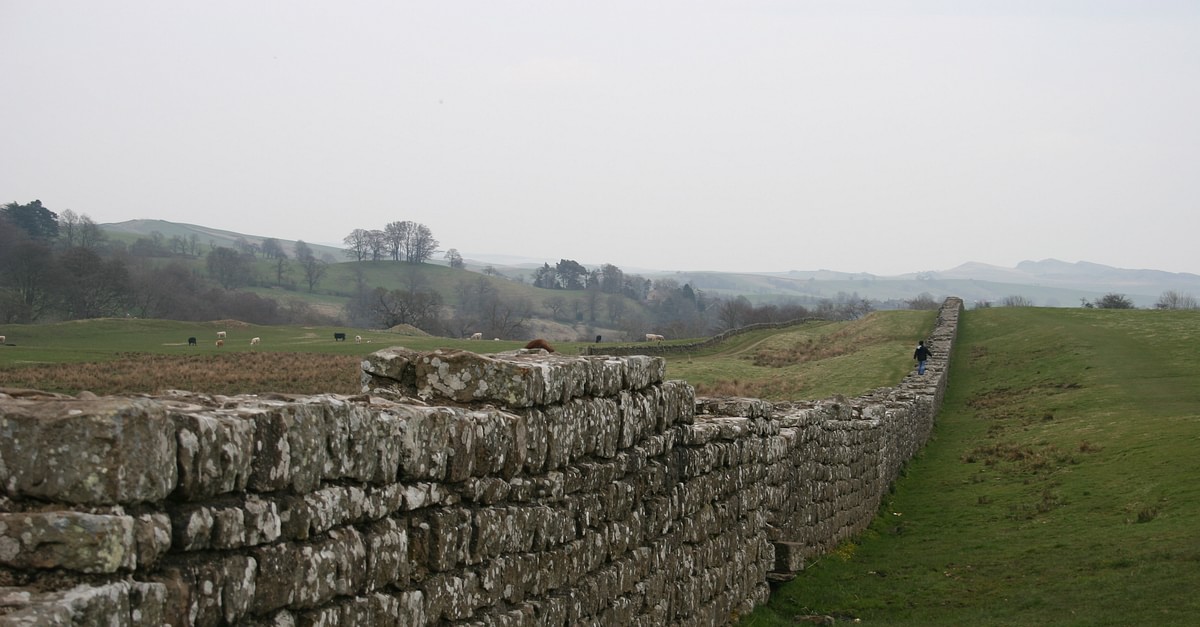This professional, detailed photograph captures an ancient stone wall stretching diagonally from the bottom left to the almost top right of the image, where it intersects with a distant mountain range. Composed of one-foot by one-foot square blocks stacked approximately six feet high, the wall exhibits signs of age with visible mold and wear from numerous rainstorms.

The landscape on either side of the wall contrasts sharply. On the left, a lush grassy field populated with various black and white farm animals extends towards light hills dotted with trees. In the background, a few scattered houses suggest a rural village environment. As the elevation changes, the grassy hills rise, adding depth and complexity to the left side of the scene.

On the right side, the terrain is flat and covered with lush green grass but devoid of animals, with only sparse foliage visible. A lone figure, a child dressed in a black coat and hat with blue jeans, walks alongside the wall in the distance, adding a sense of scale and human presence to the vastness of the landscape.

The sky is a somber gray, indicative of a recent or impending rain, which enhances the overall mood of the image. This well-worn stone wall serves as an enduring divider of the contrasting yet equally rich pastures, offering a glimpse into the pastoral beauty and historical depth of the setting.